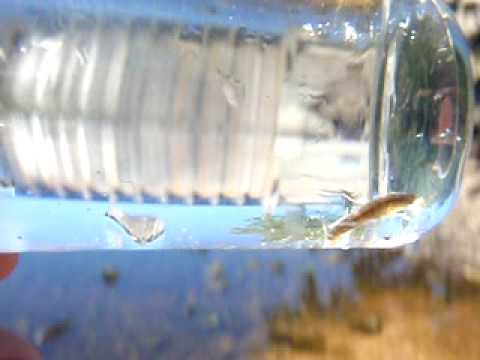The somewhat blurry image primarily depicts a horizontally-held water bottle, which could be either glass or plastic, filled with water. Inside the bottle, there appears to be a small brown object resembling a fish, positioned towards the bottom right corner of the bottle. The fish is floating amidst a lighter blue, shiny liquid, with a golden, fish-shaped object discernible at the bottle's tip. The background is fuzzy and features a mix of blue, gray, and brown, likely indicating a body of water, possibly a river or lake, with some shoreline and sand. The presence of tan and red hues adds to the varied, unclear scenery.